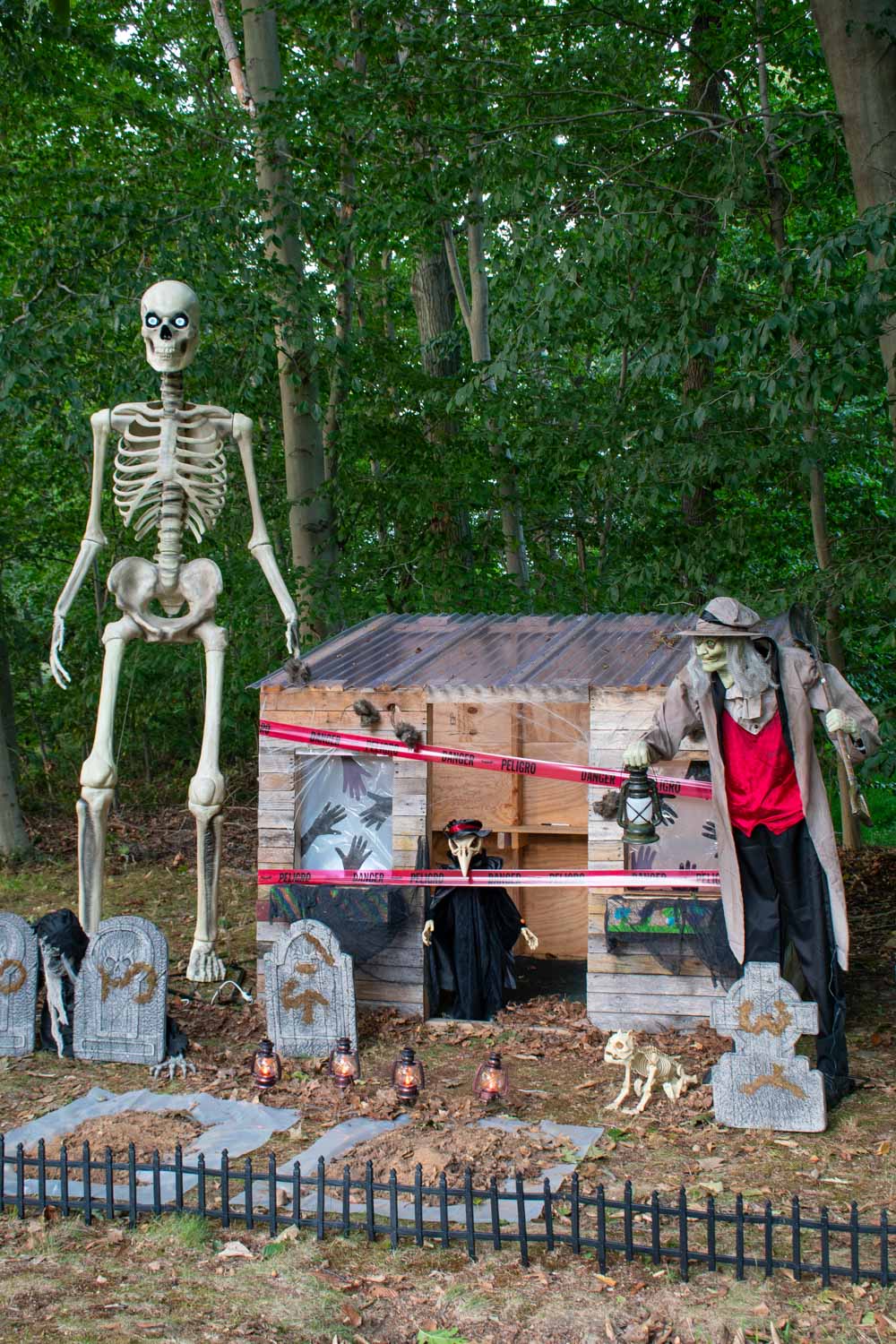In this outdoor daytime scene, the focal point is an elaborate Halloween display set up in someone's yard, surrounded by a lush, densely wooded forest that occupies the upper two-thirds of the image, with sunlight peeking through the trees. The forest floor below is scattered with leaves, dead sticks, and sparse grass.

The display features a small black fence at the front, enclosing four or five gravestones, some of which are graffitied with gold spray paint. Scattered among the headstones are small lanterns and a skeletal figure of either a cat or a dog. Dominating the left side of the scene stands a towering twelve-foot skeleton with glowing blue eyes.

Central to the display is a rustic hut with a clear plastic roof, adorned with posters and pictures. A ghoul or vampire figure dressed in a long trench coat looms at the doorway, holding a lantern and possibly a shovel. To the right, another figure, perhaps a witch, dressed in a bright red vest, black slacks, and a tan overcoat, adds to the spooky ambiance. The intricate decorations and tall skeleton against the backdrop of dense greenery create a uniquely eerie yet creative Halloween yard scene.